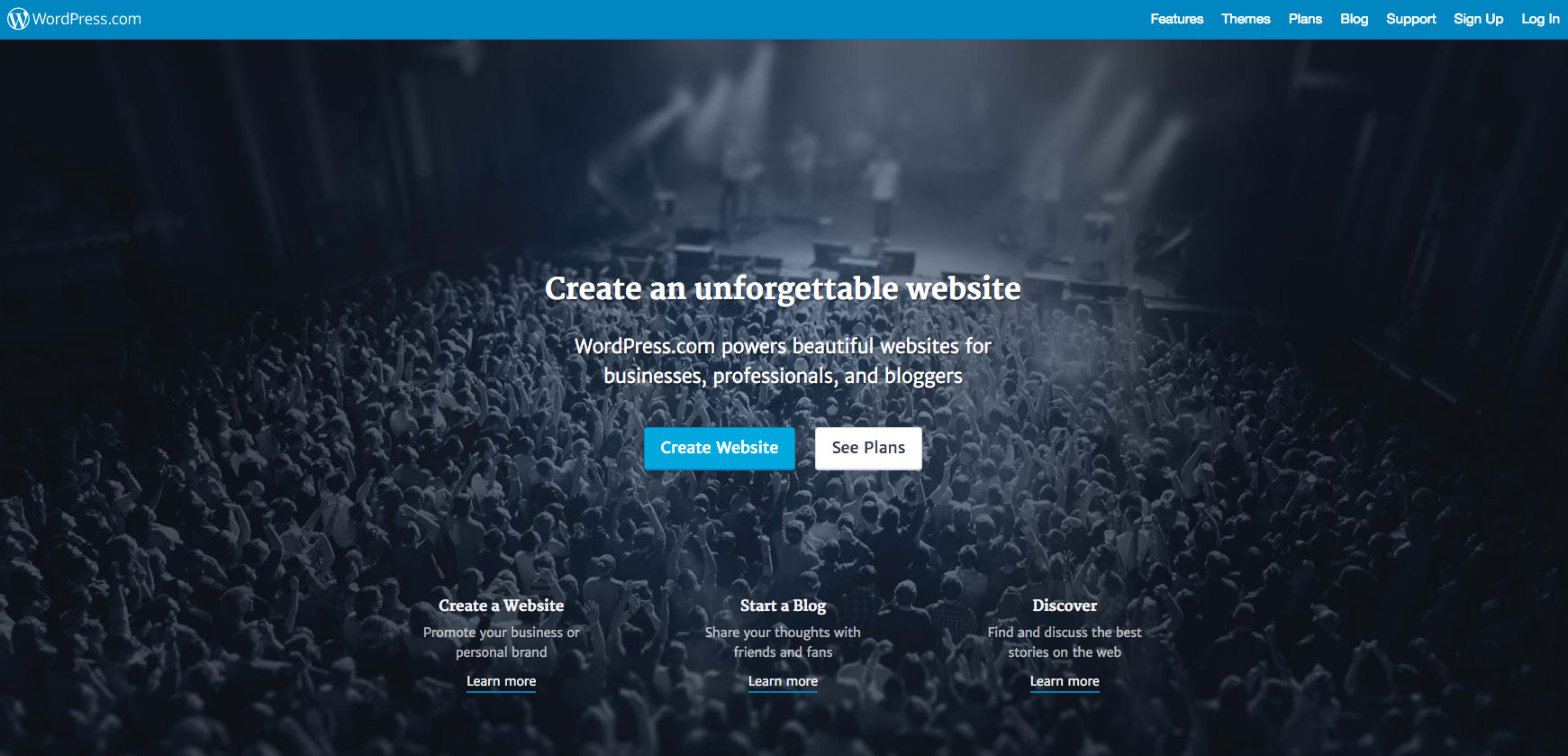This screenshot from WordPress.com features a vibrant image of a large crowd at a concert, filling the entire floor space with people standing closely side-by-side. Overlaying the image is the text, "Create an unforgettable website. WordPress.com powers beautiful websites for businesses, professionals, and bloggers." Below this, two clickable boxes are displayed: the left box is blue with the text "Create Website," and the right box is white with the text "See Plans." Further down the page, three informational sections are presented from left to right. The first section, titled "Create a Website," encourages users to promote their business or personal brand. The middle section, labeled "Start a blog," invites users to share their thoughts with friends and fans. The final section on the right, titled "Discover," suggests finding and discussing the best stories on the web.